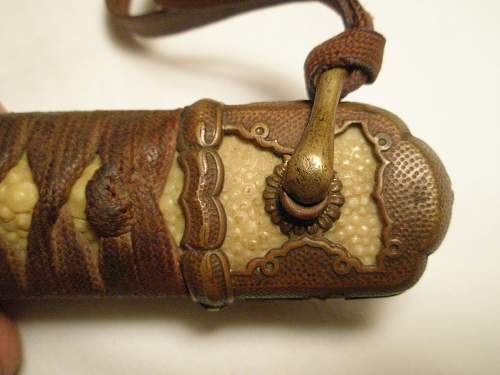This is an extremely close-up photo focusing on the end piece of an object, potentially a sword handle or its sheath, resembling something like a samurai sword holder. The visible portion of the object showcases a meticulously crafted design. The handle or sheath appears to be wrapped in a brown leather material, featuring an intricate pattern with dimples and a stylized, curved center. Exposed beneath the brown exterior is an ivory-colored segment, adorned with small circular markings. Prominently positioned in the middle of the end piece is a metal clip or clef, which has a brown string or rope attached to it, possibly for carrying. The overall composition of the image places this ornate end piece against a plain white background, highlighting the detailed craftsmanship of the leatherwork and the contrasting lighter material underneath.